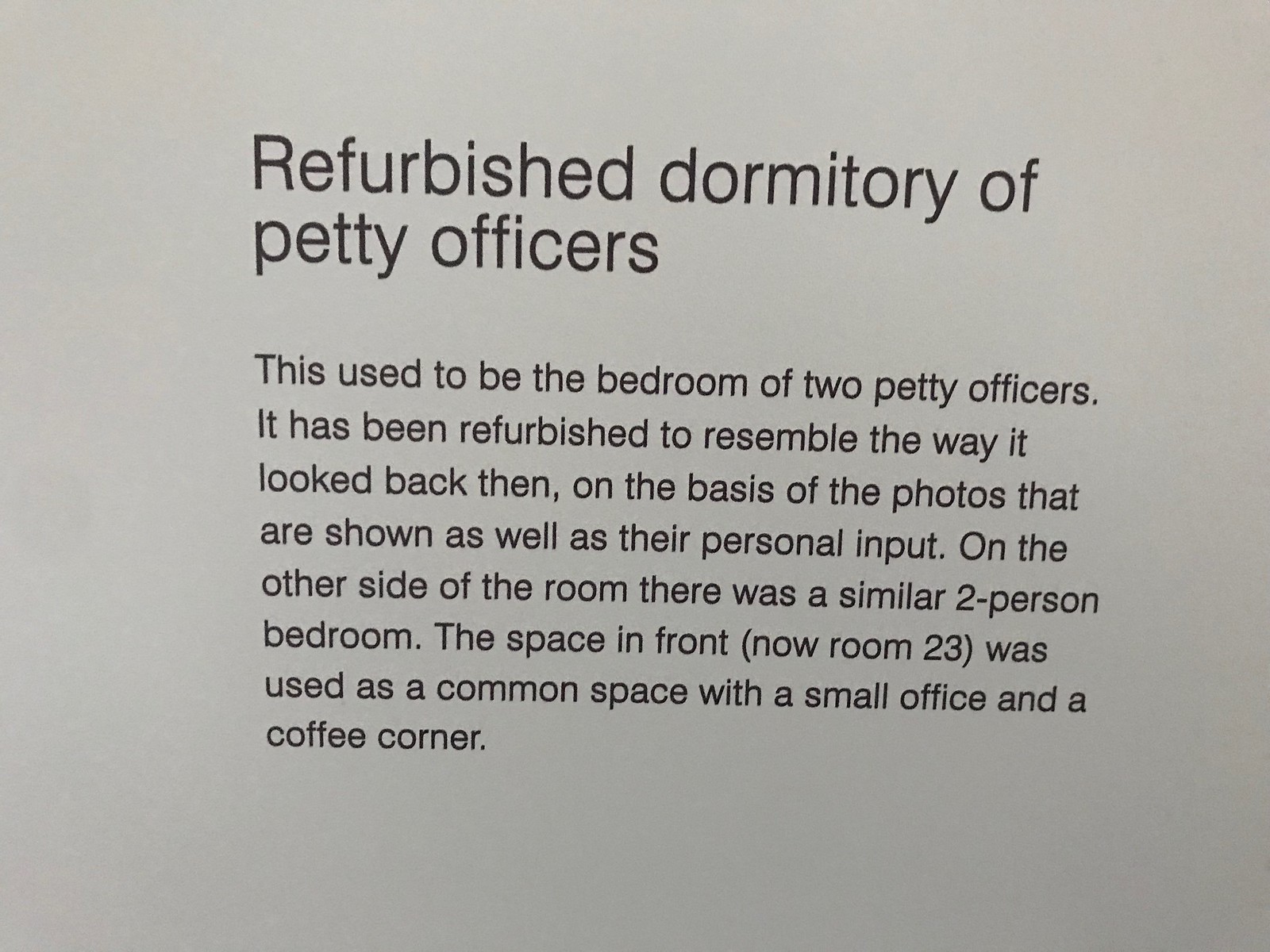The image displays a black text on a white background, likely a photograph of a sign or a printed sheet of paper. The heading in black, centered text reads, "Refurbished Dormitory of Petty Officers," with "Refurbished" on the first line and "Dormitory of Petty Officers" on the second line, but aligned as if "Refurbished" were centered. Below the heading, a centered paragraph describes the content: 

"This used to be the bedroom of two petty officers. It has been refurbished to resemble the way it looked back then, on the basis of the photos that are shown, as well as their personal input. On the other side of the room, there was a similar two-person bedroom. The space in front, now Room 23, was used as a common space with a small office and a coffee corner."

The image appears to focus on the historical refurbishment of a dormitory, providing a detailed description of how the space has been restored based on historical photographs and personal testimonies.